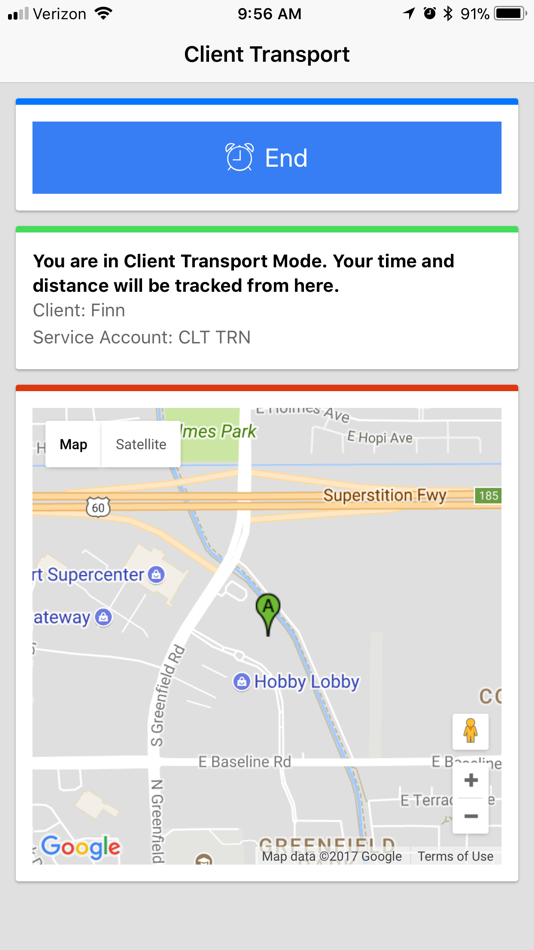The image features a gray background with several interface elements visible. In the top section, the status bar shows the time as 9:56 AM, with Verizon as the service provider and a 91% battery level. Below, an alarm clock icon is present. The center of the image displays a notification stating, "You are in client transport mode. Your time and distance will be tracked from here." 

The text indicates that the client, named FINN, is associated with a service account labeled as CLTTRN. A prominently visible blue rectangle contains the word "End" next to another alarm clock icon. 

The bottom section of the image features a map interface with two view options: "Map" and "Satellite." There is a location icon pinpointing a specific spot on the map. Adjacent to the map are various controls, including a white square with a yellow person icon, and two smaller white squares with a "+" and a "-" sign, respectively, likely representing zoom-in and zoom-out functionalities.